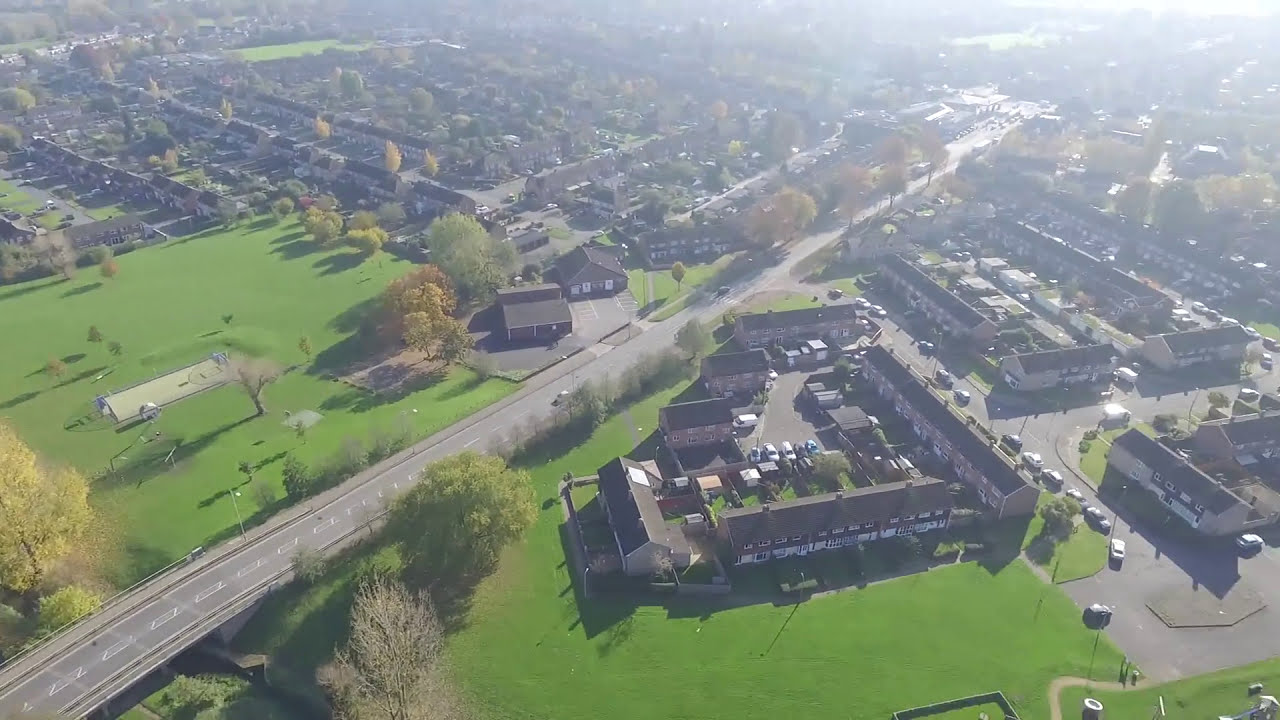This aerial photo captures a rectangular and densely populated area, featuring a mix of low-rise buildings and greenery. A prominent gray road, lined with white center stripes, stretches diagonally from the lower left corner to the upper right, dividing the image. On both sides of the road, the landscape is characterized by numerous low-rise buildings, with most appearing to be one or two stories high. These buildings have dark brown, triangular roofs and are largely rectangular in shape, resembling apartment complexes or dormitories.

To the right of the road, the structures look like long, multi-unit apartment complexes surrounded by parking lots. Many cars can be seen parked or driving near these buildings. On the left side, the buildings appear more like houses but still maintain the dense arrangement. There are also open green spaces with well-maintained grass, especially in the lower half and middle left sections of the photo, where some trees also appear to be clustered.

The overall brightness increases towards the top of the image, suggesting sunlight peeking through and casting a hazy glow over parts of the scene. The entire composition is densely packed with buildings, indicating a highly populated area without any skyscrapers, just low-rise structures across a flat landscape.